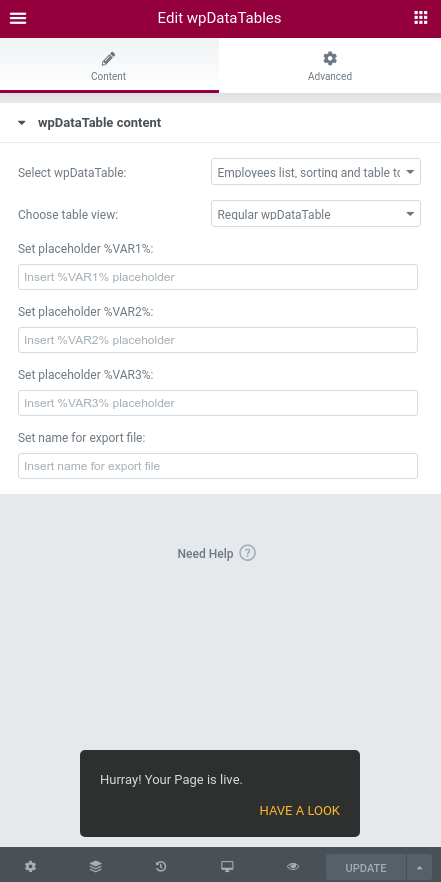In the center of the image, there's a screenshot displaying a web interface for editing WP Data Tables. At the top, the header reads "Edit WP Data Tables." There are two clickable options just below this header: the one on the left, which is currently selected, features a pencil icon with the label "Content" beneath it, while the one on the right displays a gear symbol labeled "Advanced."

Further down, the interface reiterates "WP Data Table Content" and prompts the user to "Select WP Data Table." A dropdown menu is visible, showing "Employees List Sorting and Table" as the selected option, though the rest of the text in this dropdown is cut off. Below this, the interface presents another prompt labeled "Choose Table View," with a corresponding dropdown menu set to "Regular WP Data Table."

Underneath, there are various placeholder settings: "Set Placeholder Percent, VAR 1%," "Set Placeholder Percent, VAR 2%," and "Set Placeholder Percent, VAR 3%," followed by a field labeled "Set Name for Export File." Centrally located is a "Need Help?" section featuring a gray question mark icon.

At the very bottom of the interface, a small pop-up message in the center declares, "Hooray! Your page is live." In the bottom right corner of this pop-up, there's a clickable option to "Have a Look." Along the lower edge of the screenshot, various symbols are shown alongside a dropdown menu labeled "Update."